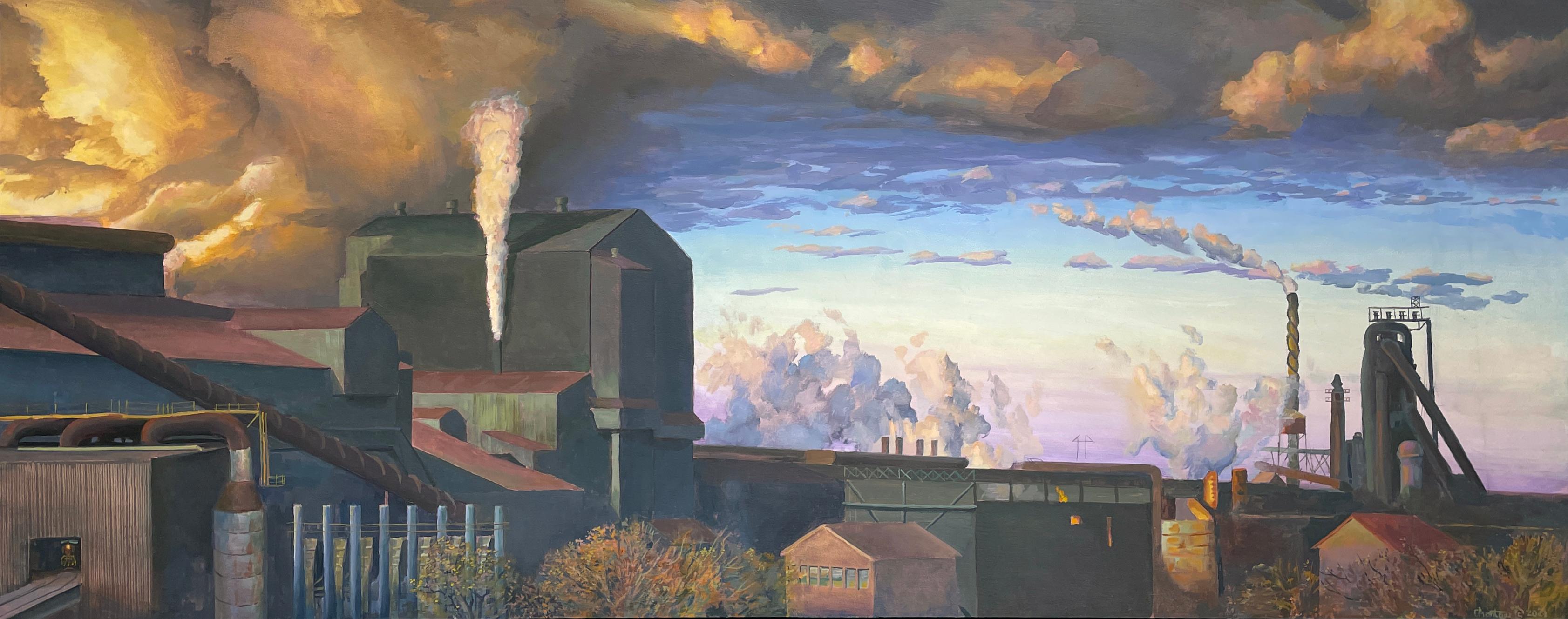This detailed oil painting illustrates a sprawling industrial town or factory primarily composed of dark brown, blue, and gray buildings clustered closely together. The buildings are equipped with multiple chimneys, from which smoke billows out, contributing to the heavy, ominous clouds overhead. The sky is a gradient of colors, with blue and yellow-white hues on the right and left sides respectively, transitioning into pinks, purples, oranges, and browns due to the industrial pollution. On the ground, there are various tools, machines, and pipes snaking around the buildings, with noticeable silver test tube-like bars. A small wooden building with an attached furnace is present in the bottom left corner. Sparse bushes, seemingly dead and reflective of a winter setting, and autumn-colored trees are scattered around in the foreground. The painting vividly contrasts the pleasant, serene sky in the distance with the dark, polluted atmosphere closer to the viewer, emphasizing the industrial activity's impact on the environment.